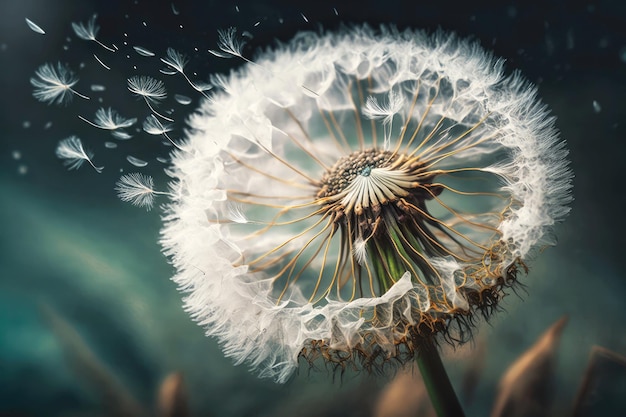This is a close-up photograph of a dried dandelion outdoors, with its seeds dispersing into the air. The image beautifully captures the intricate details of the dandelion's white seedlets, many of which are detaching from the dried center and floating towards the top left-hand corner, driven by the wind like tiny parasails. The central stalk is dry, and both the outer petals and the faded brown and green stamen or pistil can be prominently seen, with a small blue-green dot accentuating the center of the dandelion. The photo's background is a mix of dark blue-green and brown hues, creating a contrasting backdrop that highlights the delicate transition of the dandelion from flower to seed. While the lower left-hand corner of the image appears out of focus, the overall composition is horizontal, slightly longer than it is tall, providing an immersive view of this fleeting natural moment.